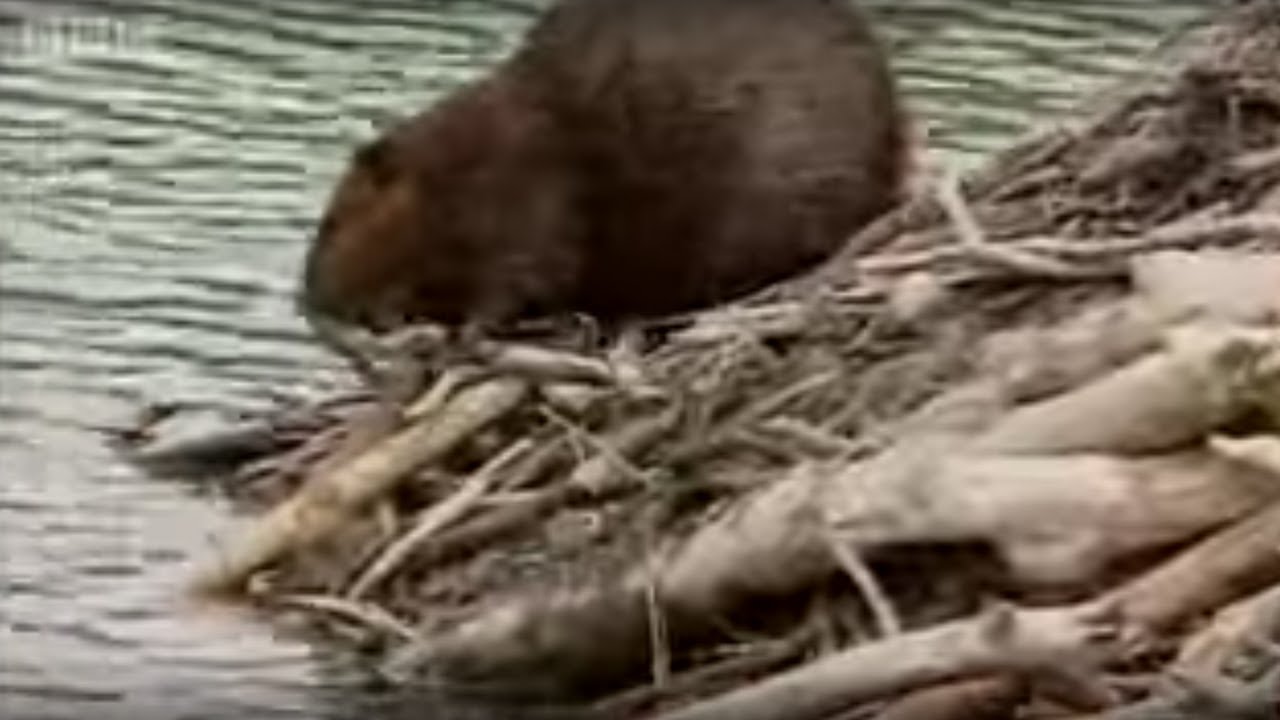In this outdoor photograph, though somewhat blurry, a brown beaver is centrally positioned, facing the water with its rear end to the right and head to the left. The beaver is situated on a mix of tree roots and limbs, characteristic of a beaver dam, which spans from the top right to the bottom right of the image. The water, a grayish-blue in color, occupies the bottom left and top left portions of the photograph. Despite the lack of text or distinct detail, the natural setting clearly depicts the beaver amid its dam construction by a river or stream, providing a scene rich with earthy browns and subtle water hues.